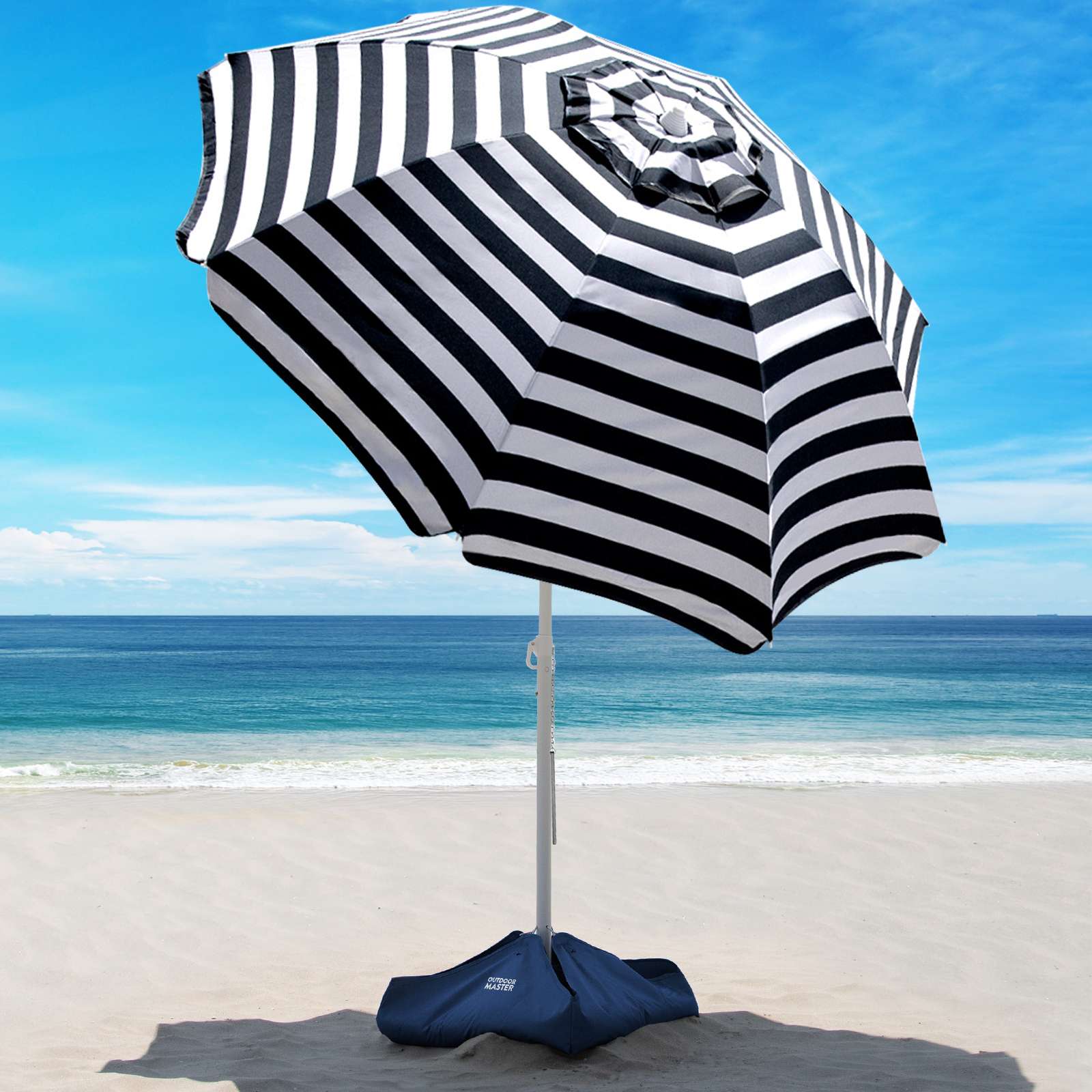This image showcases a serene, unpopulated beach with fine, pale tan sand, and a vibrant blue sky dotted with a few distant clouds. At the center of the scene is a striking navy and white striped sun umbrella with a white pole. A weight at the base ensures it remains steadfast against any breeze. The umbrella is angled towards the sun, casting a pronounced shadow on the smooth sand below. The beach itself meets a calm, blue-teal ocean that darkens as it stretches towards the horizon. Gentle waves, capped with strips of white foam, lap softly at the shore. The photograph, focusing primarily on the umbrella, evokes a sense of tranquility and solitude.